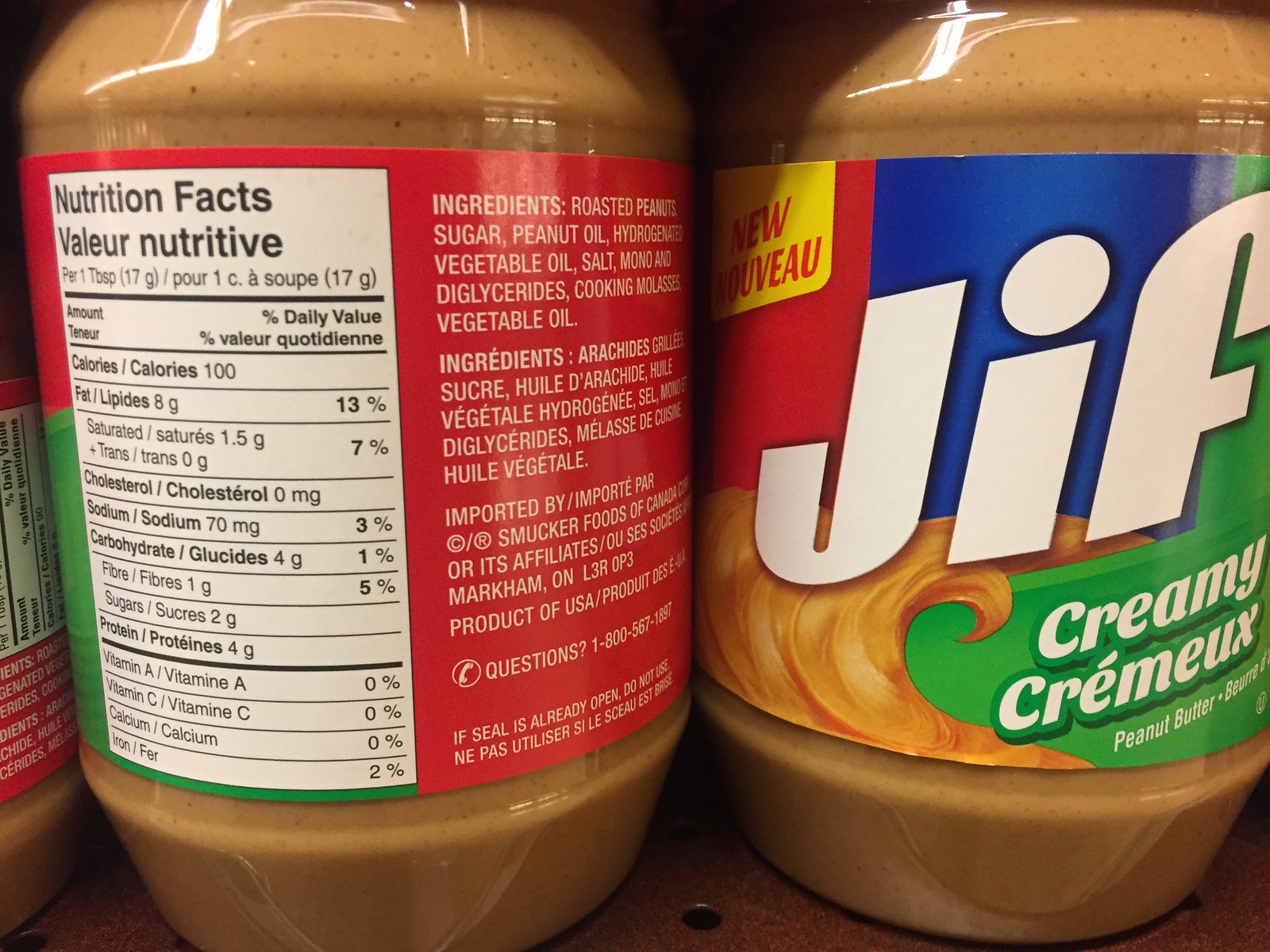This close-up image features two large jars of Jif Creamy Peanut Butter positioned on a brown shelf. The jar on the left is turned to reveal its nutrition facts label, which includes ingredients like roasted peanuts, sugar, peanut oil, hydrogenated vegetable oil, salt, mono-andiglycerides, cooking molasses, and more. This label is in a white rectangular shape and also has an address for Smucker Food Company, along with a phone number (1-800-567-1897). Some of the text appears to be in French, and it indicates that this product is made in the USA. The jar on the right prominently displays the iconic Jif logo with bold, thick letters in red and blue stripes. Below that, the label features a creamy peanut butter swirl in the bottom left corner and the word "Creamy" on a green background. Both jars are marked with the word "New" on the label. The visually rich labels and clear branding make these peanut butter jars stand out on the otherwise plain shelf.